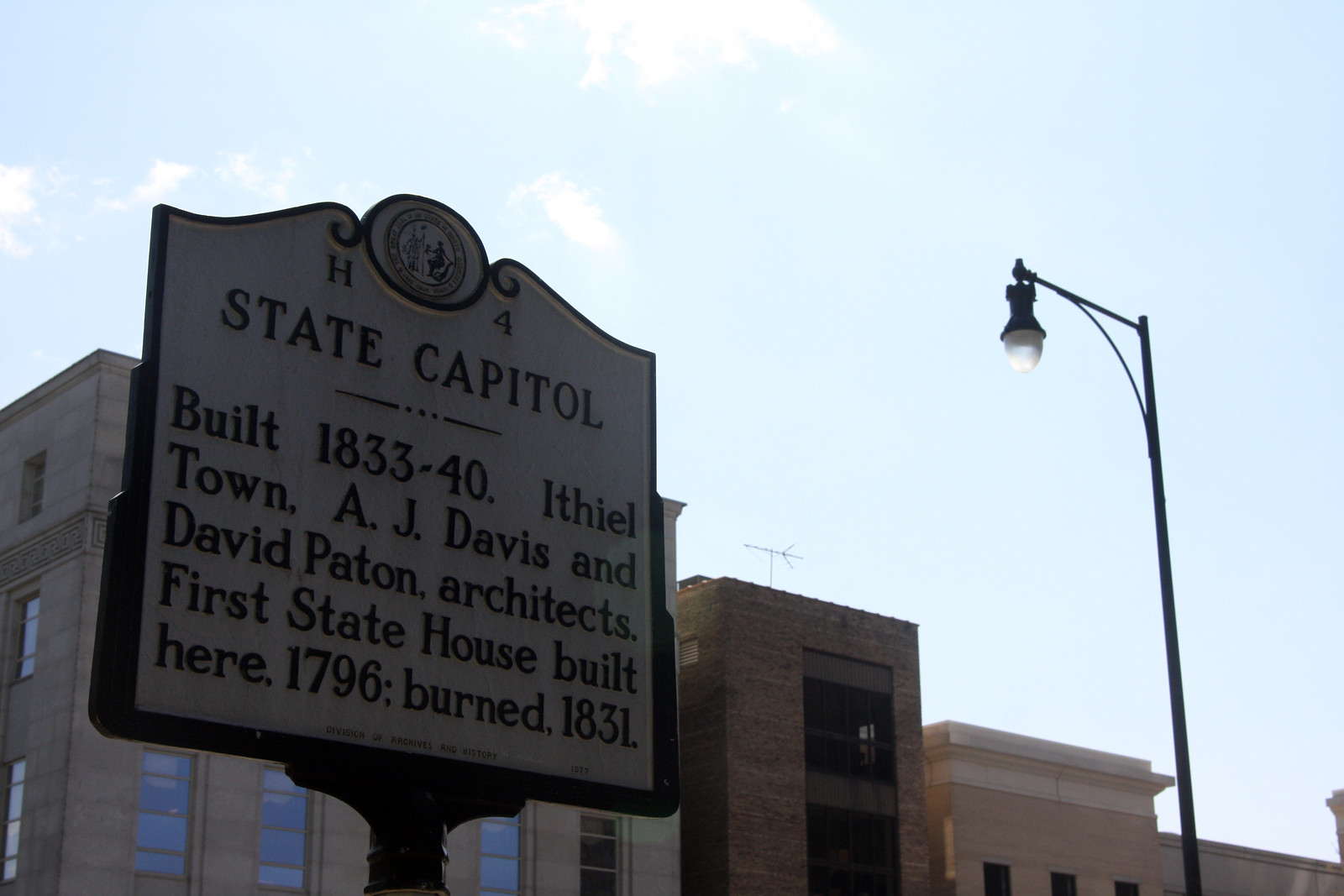The image captures a vibrant street scene featuring an old historical marker affixed to a black metal pole, positioned on the left side. The sign, designed with a white background and black ornate trim resembling the shape of a book page, bears a city crest at the top and provides detailed historical information. It reads: "State Capitol, built 1833-40, Ifealton, A.J. Davis and David Payton architects. First State House built here 1796, Burned 1831." To the right stands a tall black lamppost with an elegant globe light extending from a horizontal arm. In the background, there are beach residential buildings, displaying a mix of gray cement and red brick facades, complete with glass windows and balconies. Above, the sky is a bright blue, scattered with some white clouds, and bathed in strong sunlight, indicating a clear, bright day.